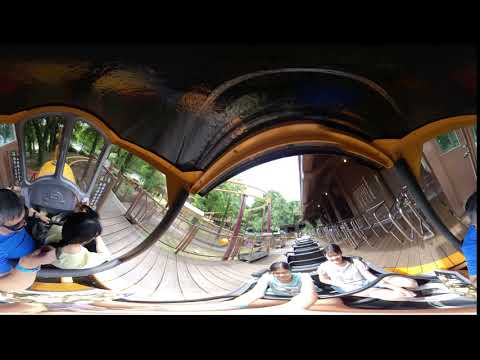In this distorted panoramic image of an amusement park ride taken during the day, we see two girls strapped into the front row of a roller coaster, positioned towards the bottom right. They are just leaving the wooden boarding gate, which features a wooden overhang and metal dividers. The roller coaster track, partially visible, leads them out into a brightly lit outdoor area. The panorama creates a warped effect, splitting a man in a blue shirt with a camera between the left and right sides of the image. Behind the girls, you can see several trees in the distance, with the sky peeking through the center. The scene includes various colors: black, silver, gold, brown, yellow, blue, light blue, and green. The image captures the excitement and setting of the amusement park, with the wooden walkway and possible metal benches enhancing the environment's lively atmosphere.